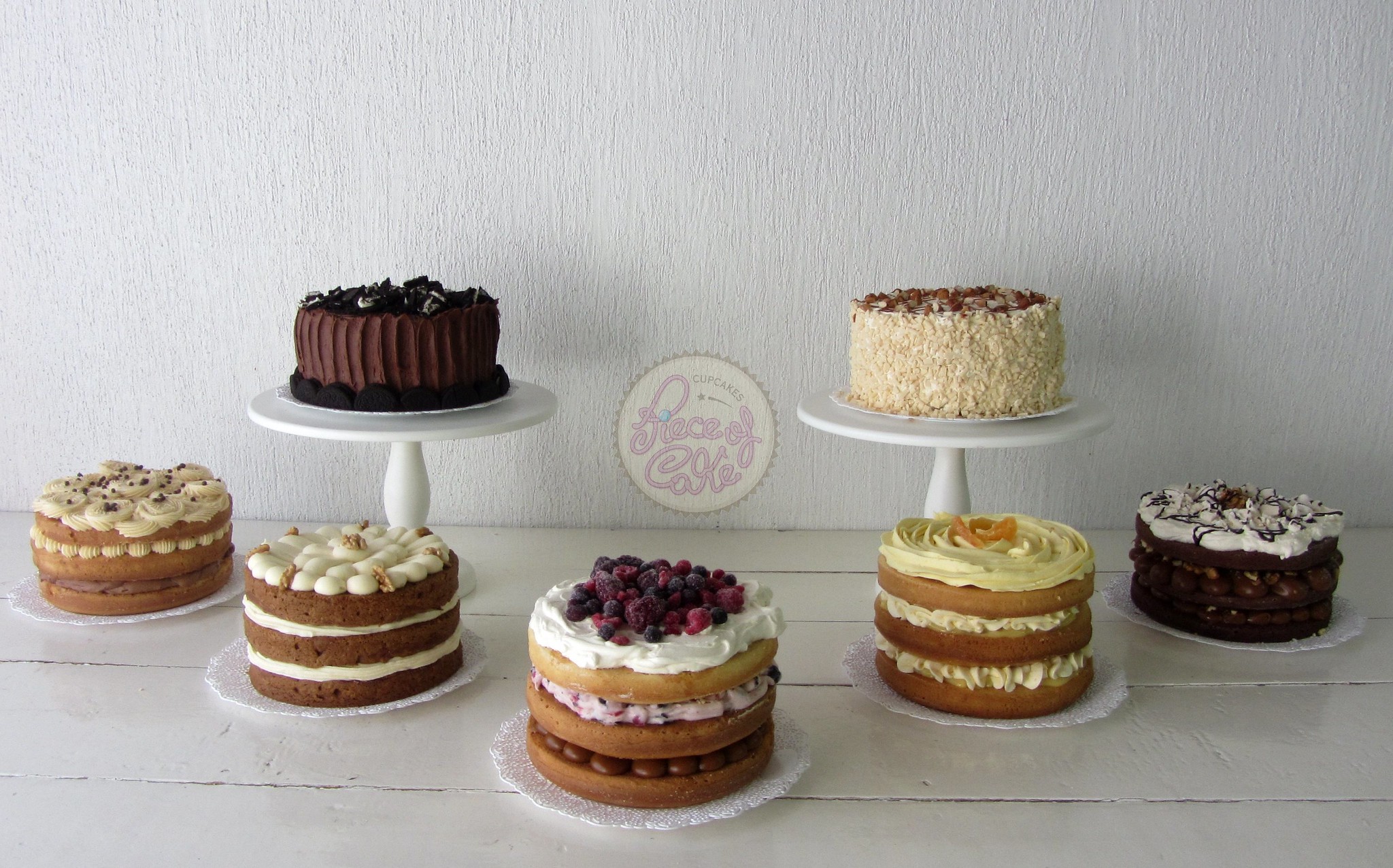This photograph features a stylish display of several types of layer cakes against a textured off-white wall. A sleek white wooden table in the foreground holds a total of seven cakes arranged in a triangular or V-like formation. Center stage, there's a plaque on the back wall stating "Piece of Cake," hinting at the name of the cake maker.

At the back of the display stand two elevated white cake pedestals. The pedestal on the left cradles a chocolate cake with rich chocolate icing, while the one on the right showcases a white cake adorned with what looks like crushed brown toppings.

In the foreground, five cakes are meticulously arranged, each on a white plate. Starting from the upper left, the first cake is a two-layer creation with exposed sides and a generous layer of white icing on top. Just below it, a three-layer cake also flaunts white icing. In the center, a three-layer cake garnished with mixed berries adds a splash of vibrant color. Up to the right, a three-layer cake boasts yellow icing and is adorned with small orange slices. Lastly, the cake in the upper right corner is a decadent chocolate creation with white icing and a graceful drizzle of chocolate on top.

Each cake is uniquely decorated, showcasing a variety of icings and toppings that provide a visual feast for the eyes, perfectly complementing the rustic yet elegant setting.